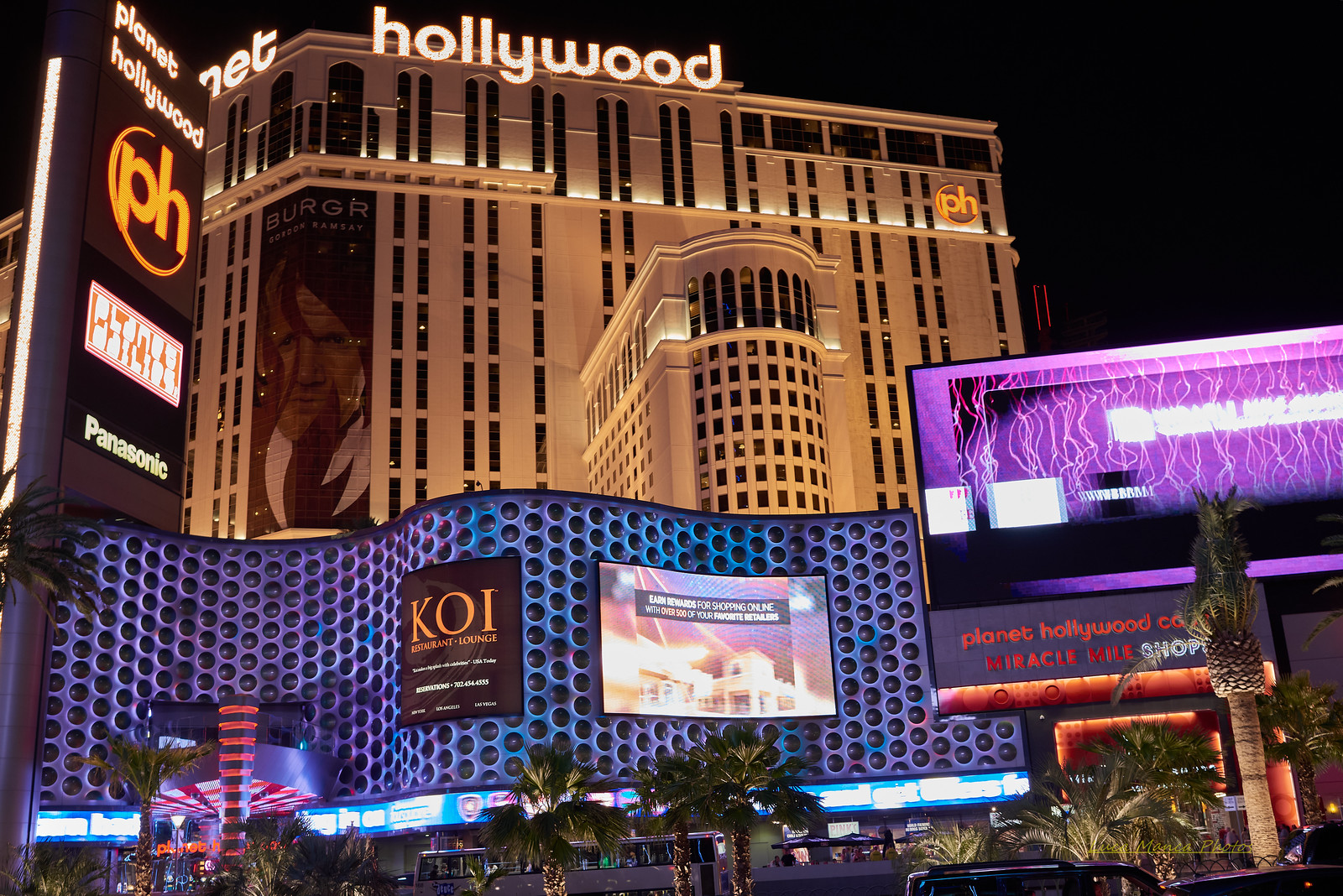The image showcases a brightly illuminated downtown nightscape with a dominant tall, gold-colored building that displays the name "Hollywood" in glowing white letters at the top, suggesting an ambiance akin to Las Vegas. Below this prominent structure, the bustling street is lined with various vibrantly lit signs and buildings. On the left, a large black billboard for "Planet Hollywood" features a striking orange PH symbol and the word "Panasonic" underneath. Nearby, another detailed rectangular sign advertises "Planet Hollywood Miracle Mile Shop" in purple hues, adding to the dynamic color palette. Amongst the architecture, several palm trees add a touch of nature while blending into the vibrant scene of blues, purples, and turquoise, possibly changing colors due to the lights. Numerous display screens are visible, including one promoting KOI Restaurant Lounge and another showing an abstract image. Vehicles, including a bus and two cars, traverse the road below, adding to the lively, energetic atmosphere of this urban setting. A smaller part of the scene reveals a curved wall-like structure with multiple displays, further contributing to the bustling and vibrant feel of the area. Overall, the photo captures a vivid and detailed nighttime view of a city replete with iconic signage and modern lighting.